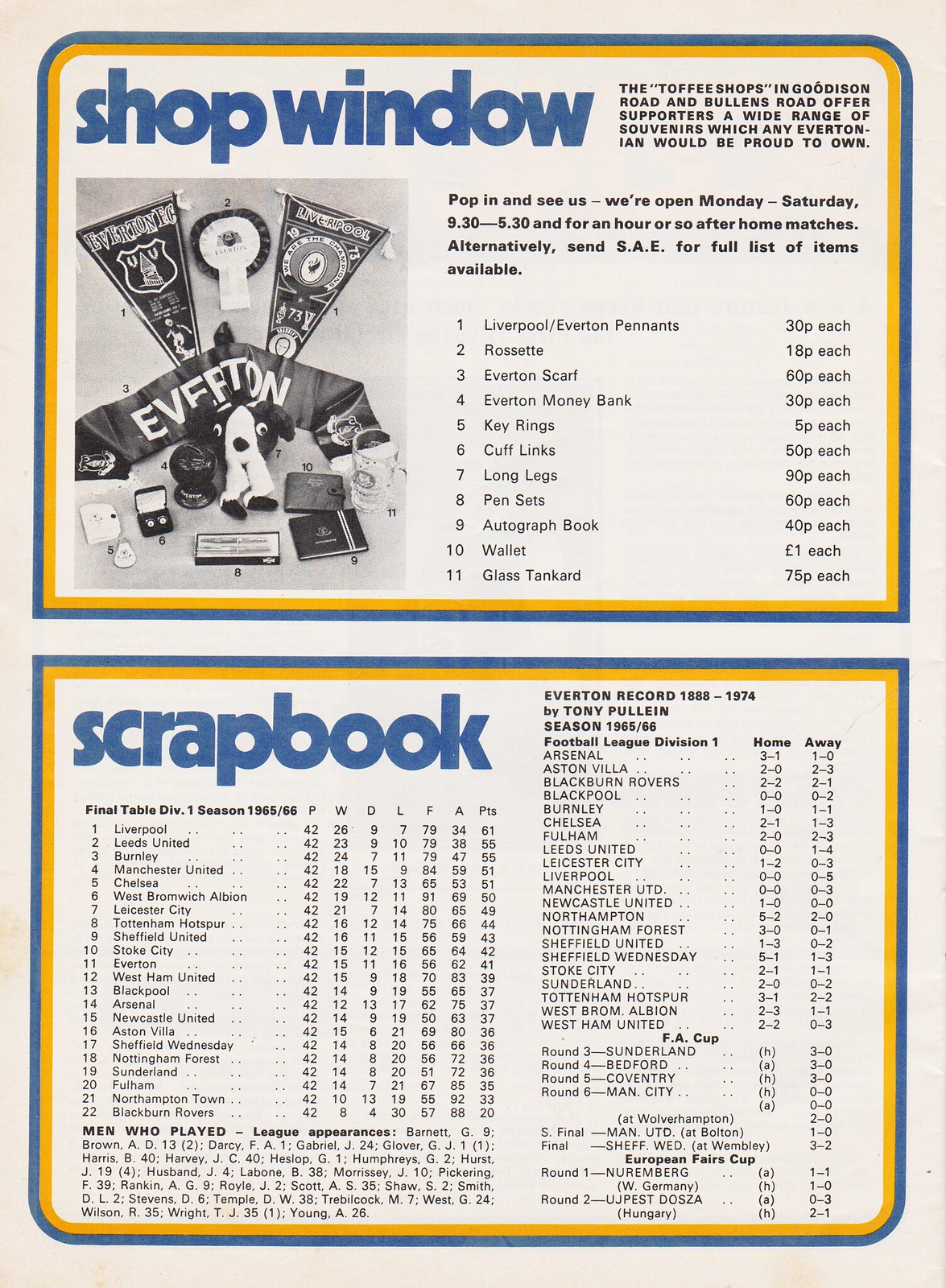This image is an advertisement from a soccer or football club program dating back to around 1974. The page, in portrait orientation with light gray background, is in black and white with spot color in dark blue and gold. It is divided into two half-page sections, each outlined with blue and gold rules with curved corners.

The top half features the heading "Shop Window" in bold dark blue letters on the left. Adjacent to the heading, there is a black-and-white photograph showcasing pennants, banners, and various sports memorabilia. Next to the photograph, a paragraph in black text describes an Everton-focused shop that offers a wide range of souvenirs, emphasizing items like Liverpool Everton pennants, rosettes, scarves, money banks, keyrings, cufflinks, pen sets, autograph books, wallets, and glass tankards. The text encourages supporters to visit the shops located on Goodison Road and Bullens Road, highlighting operating hours from 9:30 AM to 5:30 PM, Monday through Saturday, and for an hour after home matches. It also mentions an option to send a self-addressed envelope (SAE) to receive a full list of available items.

The bottom half of the page is similar in format but labeled "Scrapbook" in bold blue letters. This section contains detailed columns and rows of statistics and records, notably showcasing the final season scores for 1965-66 and other team and player statistics.

Overall, the advertisement effectively combines vibrant descriptors with structured formatting and vintage publication style to provide comprehensive information about the shop's offerings and operate times, alongside club records.